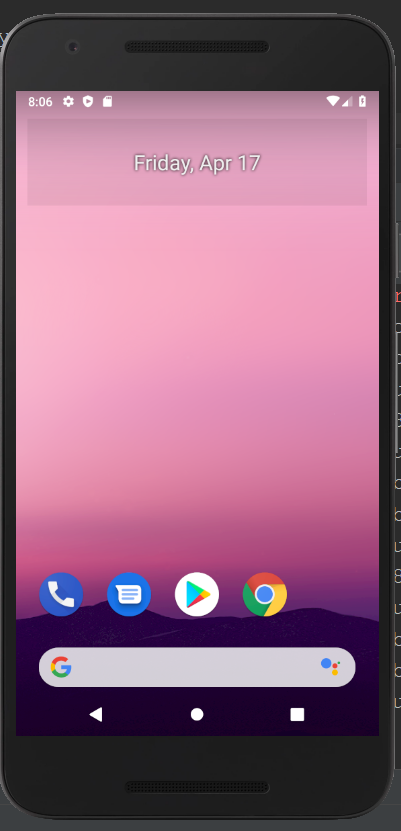The image showcases a smartphone held horizontally, revealing a web page on its screen. The phone has a black frame, and the screen itself displays a pinkish-purple background. A dark purple banner spans across the bottom of the screen. In the upper-left corner, white text reads "8:06," accompanied by various symbols. On the top right, additional icons indicate Wi-Fi strength, battery level, and other indicators.

Centrally, near the top of the page, light gray text states "Friday, Apr 17," set against the purple backdrop. Below this text, there are four ovals, which appear slightly elongated or out of shape, suggesting some distortion. The first oval on the left is blue with a phone icon. The second oval, also blue, features a message symbol. The middle oval is white and contains a blue, red, green, and yellow arrow pointing to the right. The fourth oval displays the Chrome symbol with its signature multi-colored design.

Below these ovals is an elongated, rounded rectangle with a "G" for Google on the left and several small circles on the right. Further down the page, there's a white left-pointing arrow, a circle in the center, and a small red-white rectangle beneath.